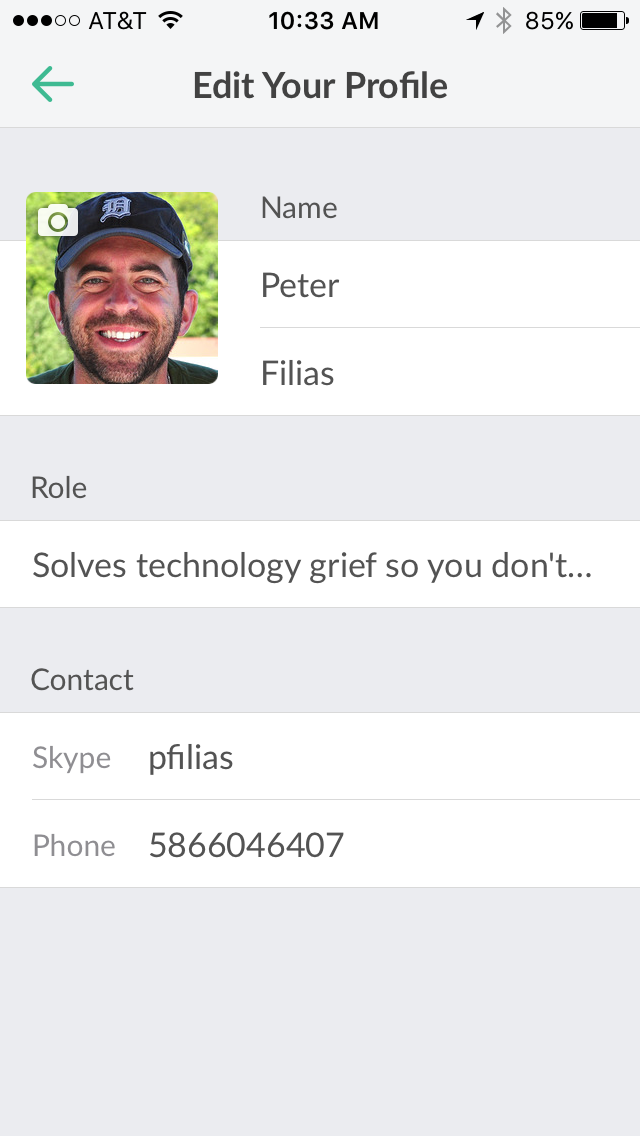The image depicts a screenshot of a mobile phone displaying an app or website in the "Edit Your Profile" section. The top status bar indicates it is 10:33 AM, connected to AT&T with full signal, and shows a battery level at 85%, along with a Wi-Fi signal icon and a greyed-out Bluetooth symbol. Underneath, a green leftward-pointing arrow appears next to the text "Edit Your Profile". The profile section features a smiling man with dark hair, a dark beard and mustache, squinting eyes, wearing a black baseball cap with a stylized letter "D" and a black shirt. The profile picture shows a background of blurred leaves. To the right of the picture, the name "Peter Filias" is listed, followed by the role description "Solve technology grief so you don't…". The contact section below includes "Skype: P. Filias" and "Phone: 586-604-6407". The fields containing user information are white, whereas the background is gray. An additional camera icon is visible at the top left of the profile image.